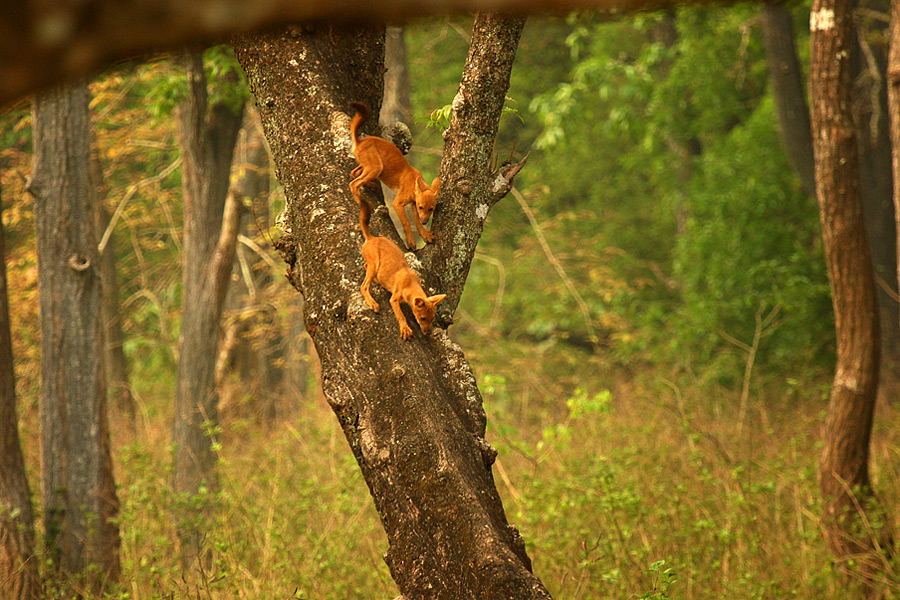The photograph captures two young, orange-colored animals perched in the crook of an old-growth oak tree, roughly five to six feet off the ground. Their unique physique combines traits of dogs, foxes, and young deer, with slender, elongated faces reminiscent of Siamese cats or hairless cats. The animals, potentially puppies or cubs, are engaging in playful activity, one actively climbing down while the other looks downward. The oak's bark is adorned with moss, and its trunk grows slightly left of center with a prominent branch extending at a 45-degree angle. The setting is a forest during the daytime, featuring vibrant green leaves and mid-waist-high grasses. Numerous tree trunks are visible in the background, emphasizing the dense woodland environment. The animals' golden fur is predominantly uniform, except for hints of black on their tails.